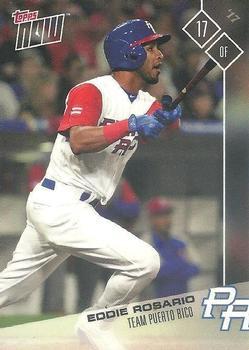This is an image of a Topps Now baseball card featuring Eddie Rosario, an outfielder for Team Puerto Rico. The card prominently displays the Topps Now logo in the top left corner, with "Topps" in a red font. In the upper right, there is a diamond containing a lightly colored number 17 and the letters "OF" indicating his position as outfielder, with a white line extending from the diamond to the bottom right corner, where it intersects with a “PR” logo representing Puerto Rico. Eddie Rosario is pictured mid-swing, appearing as if he’s just made contact with the ball and is preparing to run. He is dressed in a white jersey with red sleeves, blue gloves, and a blue helmet featuring a red brim. He also sports a red wristband. At the bottom of the card, his name, "Eddie Rosario," and "Team Puerto Rico" are printed in black text. Faintly in the background, fans and figures likely to be coaches are visible, adding depth to the image. This card, numbered 17, is a testament to his representation of Puerto Rico in baseball.